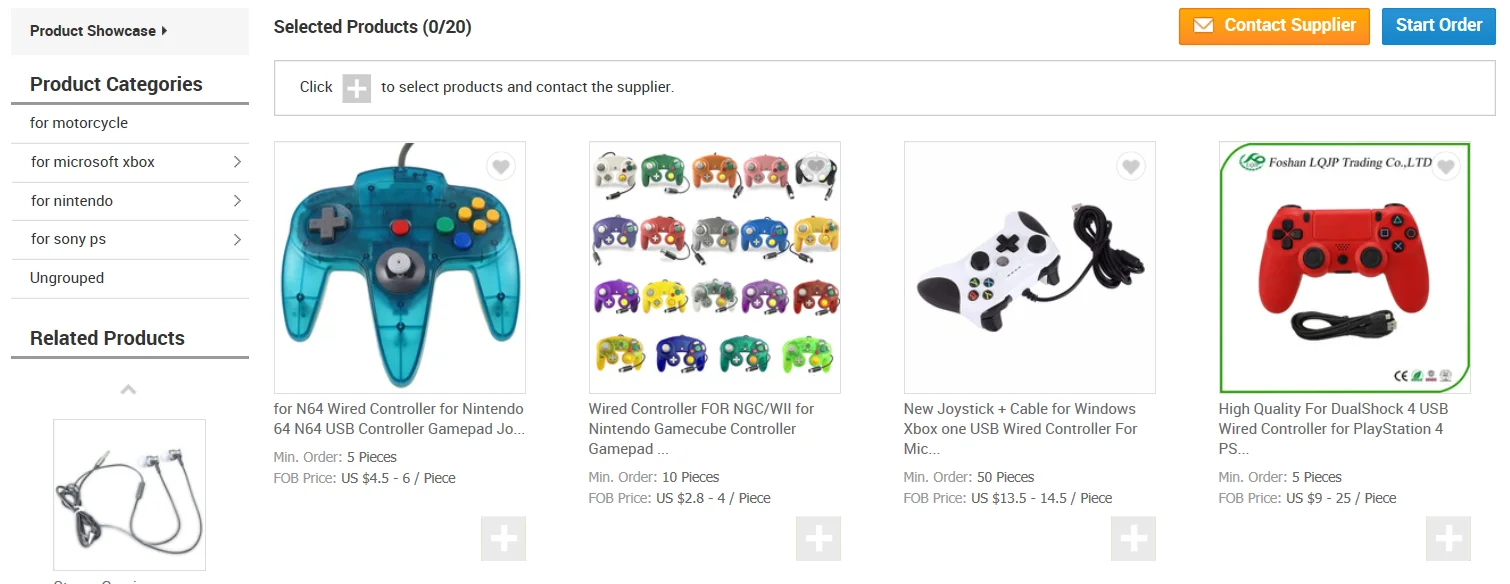This image captures a partial screenshot of an e-commerce website, specifically showcasing a product page for video game controllers. The snapshot is a rectangular cut that only includes the middle section of the web page, eliminating both the URL bar and the bottom portion of the page, suggesting it's taken from a desktop view.

The website has a clean, white background. On the left side of the screenshot, there is a vertical column offering navigation through various product categories. Adjacent to this, a header reads "Selected Products, 0 out of 20," indicating a selection feature for multiple items. Below this, the main content area displays four images of different video game controllers available for purchase:

1. **Nintendo 64 Style Controller**: A blue, translucent controller featuring a classic design with a single joystick, a D-pad on the left, and brightly colored buttons in yellow, green, blue, and red.

2. **10-Pack of Nintendo GameCube and Wii Controllers**: Despite the description stating a 10-pack, the image showcases 20 controllers, arranged in a compact manner to fit the frame.

3. **Xbox One Wired Controller**: This product is characterized by a sleek white and black color scheme, illustrating a modern and ergonomic design tailored for Xbox One.

4. **PlayStation 4 DualShock USB Wired Controller**: A vibrant red controller with contrasting black buttons, representing the iconic DualShock design specific to the PlayStation 4.

The screenshot serves as a glimpse into a shopping interface specifically targeting video game enthusiasts.